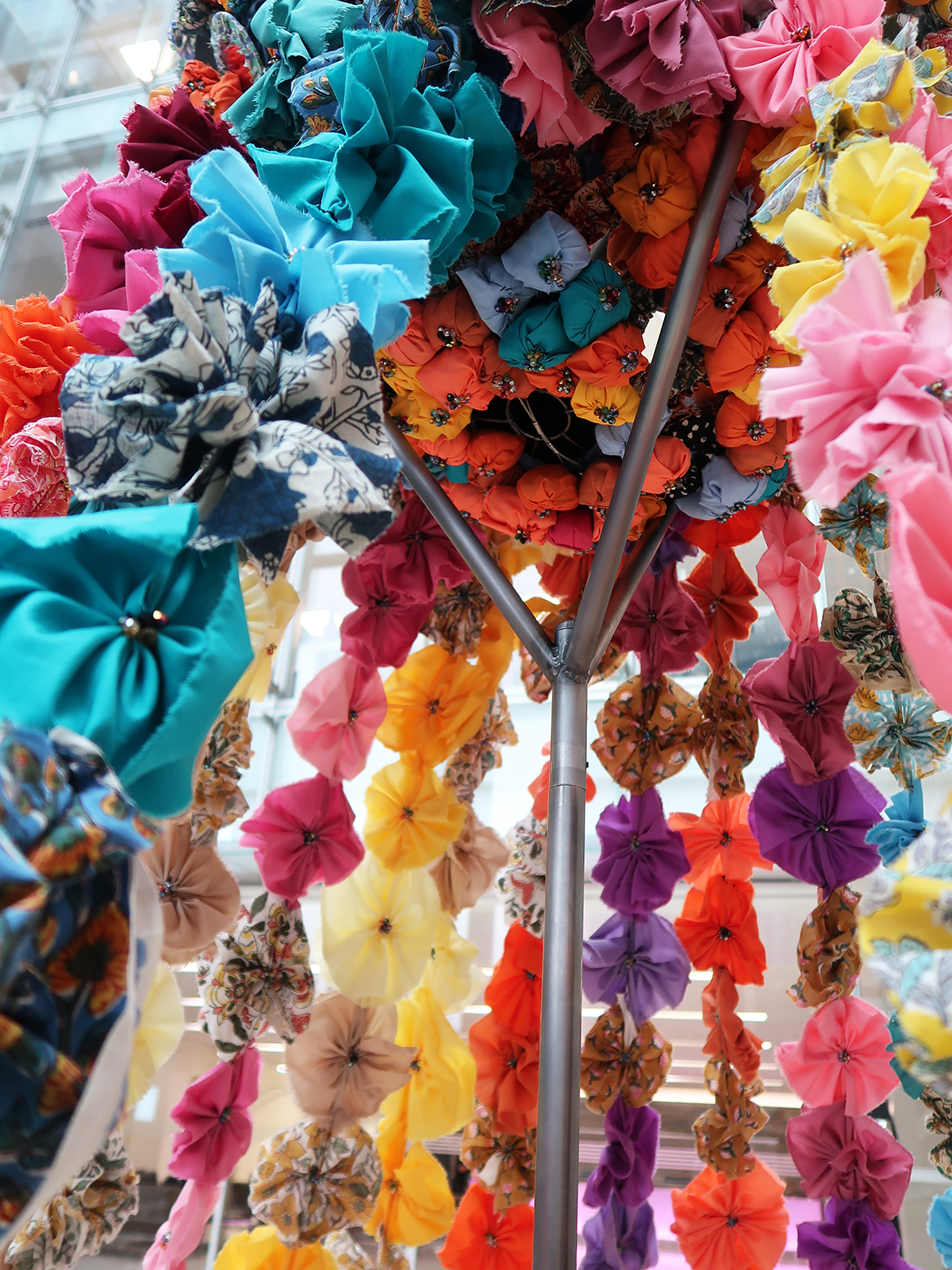The image depicts an array of delicate, cloth flowers, meticulously pinched in the center with pins to resemble small, colorful blossoms. These faux flowers, featuring hues of purple, pink, brown, yellow, orange, green, light blue, dark blue with gold prints, and multicolored patterns, are arranged vertically and appear to be suspended along strings. They cascade from a central metal device, where a long silver rod branches out into three directions—back, right, and left—providing support for the hanging blossoms. The flowers, displaying evident creases and folds in the fabric, bestow an enchanting charm despite their artificial nature, creating an impression of a vibrant floral tapestry. This vertical photo emphasizes their intricate and cute arrangement, with clusters of flowers densely adorning the strings from top to bottom, and prominently occupying the entire visual frame.